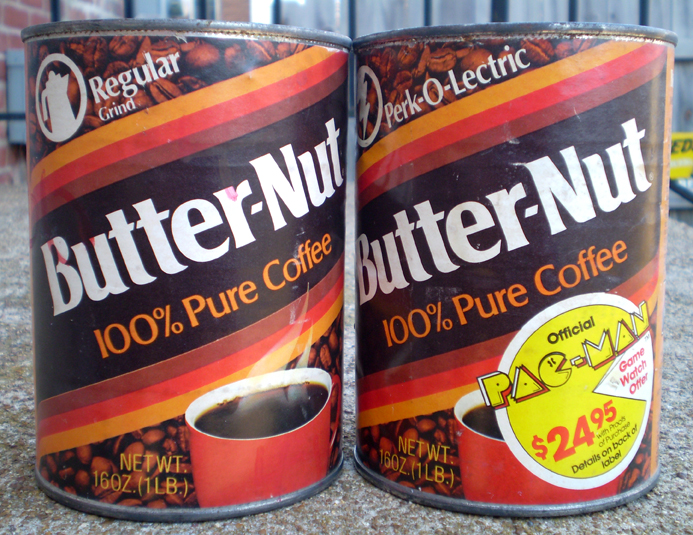This image captures two vintage 16-ounce metal cans of Butternut 100% Pure Coffee, placed on a grey cement surface outdoors. The textured ground is a small crust of gravel, and the background features weathered, faded grey wooden fence posts, suggesting an outdoor setting next to a house. 

Both cans feature a classic design with the brand name "Butternut" prominently displayed in white lettering within a dark brown section. Surrounding this central label are vibrant stripes in red, orange, and brown hues that spiral from the middle of the right side to the top left.

At the top of the cans, there's an illustration of a percolating coffee pot with the words "Regular Grind" beside it. Additionally, there are repeating striped patterns in brown, red, and yellow colors at both the bottom and top of the cans, where coffee beans are illustrated as a background.

A red coffee cup filled with steaming black coffee is illustrated at the bottom left corner of both cans. The can on the left includes an additional feature: a yellow circle with white trim and text promoting an "Official Pac-Man Game Watch Offer" for $24.95, distinctively marked by the iconic Pac-Man font.

The can on the right subtly differs as it bears the inscription "Perk-o-Electric" in the top section, differentiating it from the left. Both cans showcase a nostalgic look, presumably designed during the era when such products were common in metal cans requiring a can opener.